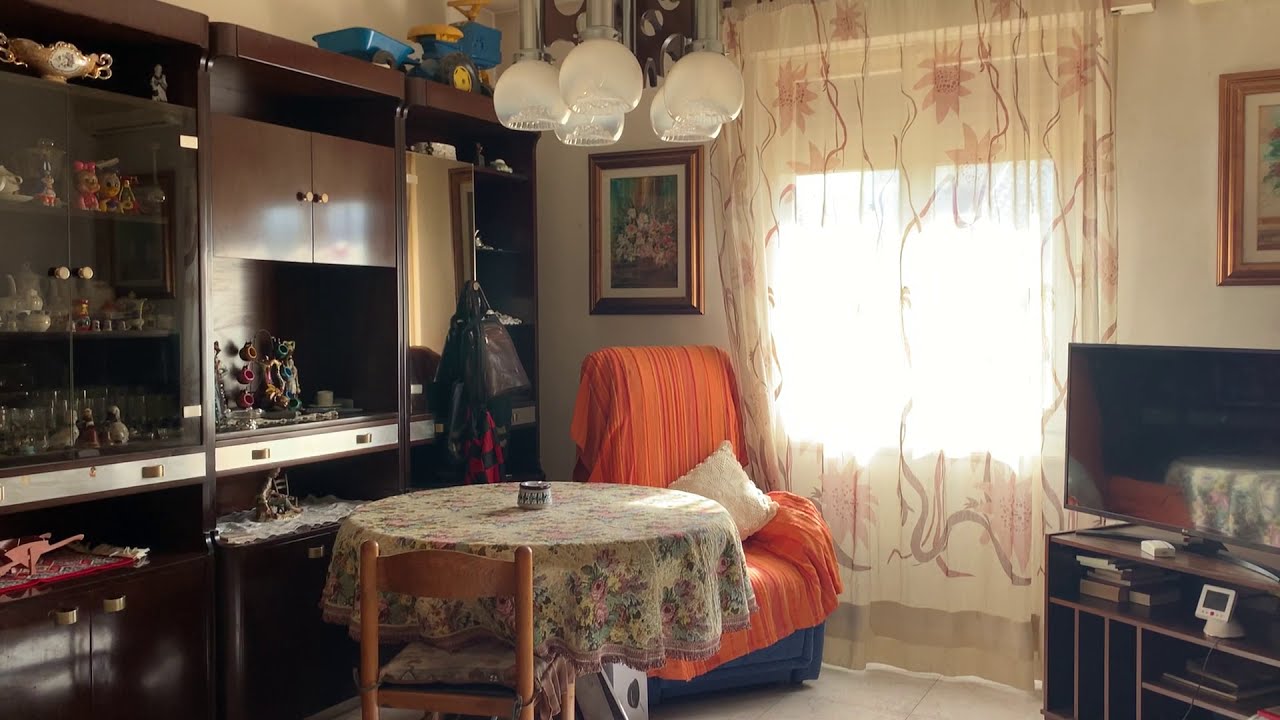This is a detailed image of a cozy, well-decorated living room corner where two off-white walls meet. The floor is laid with white tiles. On the bottom right, you see a sleek, black flat-screen TV perched on a dark brown wooden cabinet with books tucked into its shelves. Above the TV is a partially visible gold-framed painting. To the left of this frame is a large double glass door covered by sheer curtains adorned with pink flowers and green vines, allowing bright sunlight to filter through.

Prominently featured on the left side of the image is a dark brown wooden display case filled with an array of dolls, pottery, and various knick-knacks. Below the cabinet are additional storage compartments. In the center of the room, a round table is positioned, embellished with a floral tablecloth and a small bowl or pot in the middle, accompanied by a single wooden chair neatly tucked in.

Directly behind the table, a cushioned armchair draped in an orange cover and topped with a white pillow nestles close to the window. Hanging from the ceiling are five frosted and clear glass lampshades shaped like inverted cups, adding a touch of elegance to the room. Overall, the space is a harmonious blend of functionality and decorative charm, epitomizing a welcoming atmosphere.